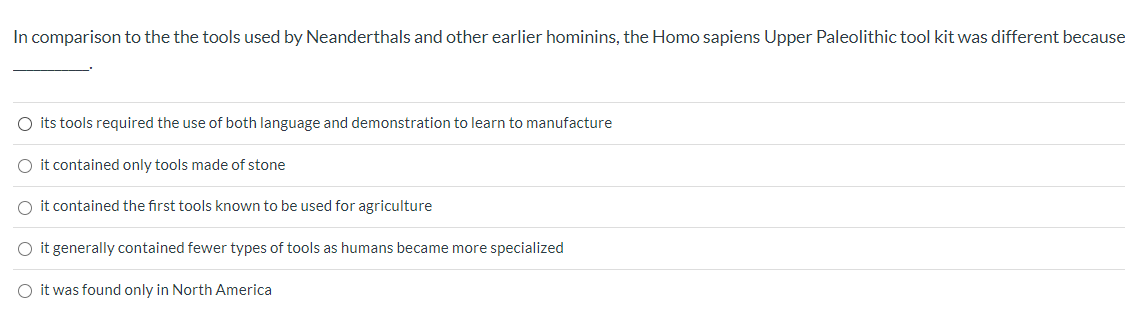A minimalistic web page is displayed, featuring a multiple-choice question likely designed for an educational test. At the top, centered in a simple, unembellished font resembling Times New Roman, the question reads: "In comparison to the tools used by Neanderthals and other earlier hominins, the Homo Sapiens Upper Paleolithic Toolkit was different because..." A blank line follows, indicating where an answer should be marked.

Below the question, five answer options are listed in a slightly smaller, more difficult-to-read font. Each option is preceded by an empty circle, indicating that respondents should select one. The options are as follows:

1. "Its tools required the use of both language and demonstration to learn to manufacture."
2. "It contained only tools made of stone."
3. "It contained the first tools known to be used for agriculture."
4. "It generally contained fewer types of tools as humans became more specialized."
5. "It was found only in North America."

Despite the minimal design, the smaller font used for the options makes readability challenging.